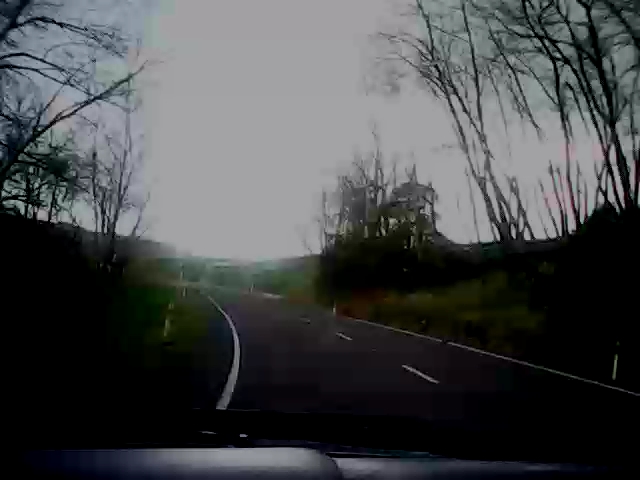This photograph, taken from inside a vehicle through the front windshield, captures a rainy daytime scene. Individual raindrops are visible on the glass, while the overcast sky appears blurred and whitewashed. Tall, nearly leafless trees line both sides of the winding road, accentuated by patches of grass. The road curves ahead with white markings along its edges and dashed lines in the center, guiding the vehicle through the turn.